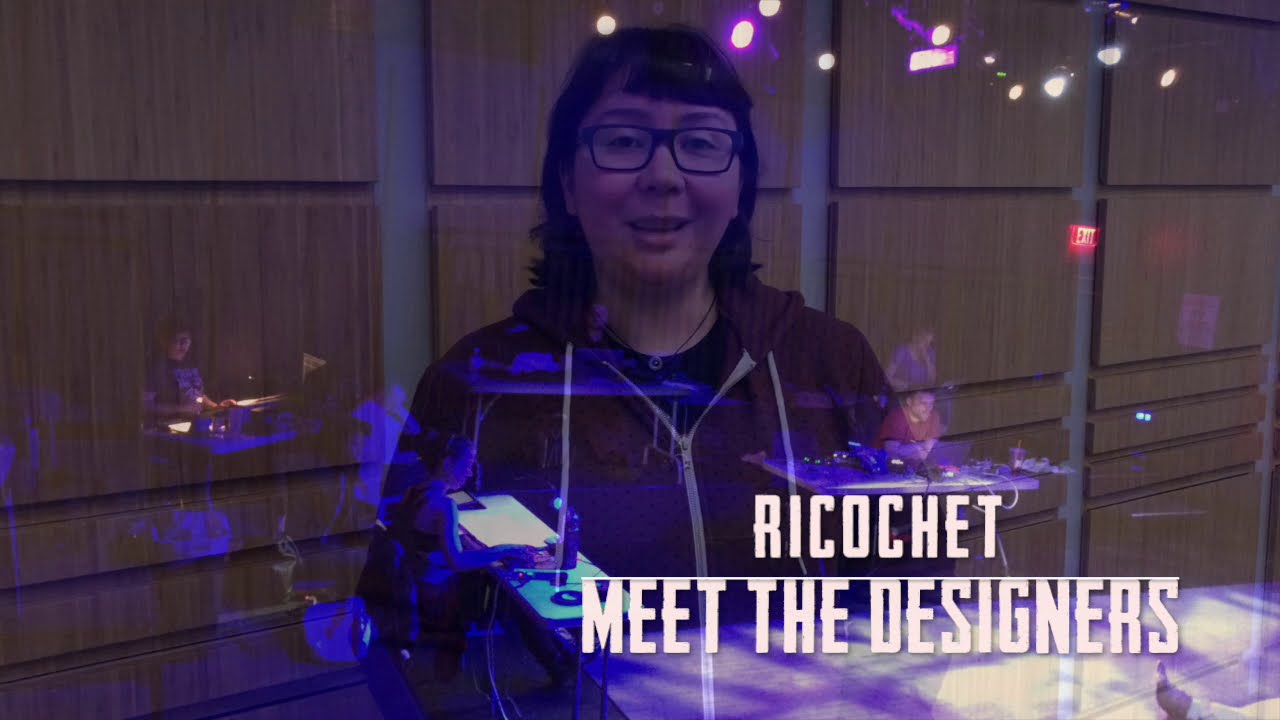This image captures a woman with black hair and glasses, faintly smiling. She is wearing a hoodie, possibly in shades of red or purple, featuring the text "Ricochet Meet the Designers" in white at the bottom. The setting appears to involve multiple layers of reflections and lights, giving a double exposure effect. The woman is seated behind a desk, surrounded by an environment with a purple ambiance. Other elements in the picture include people seated at tables working on computers, one of which is a man. The image also shows various patterns on the wall, contributing to the overall reflective and somewhat illusionary composition.